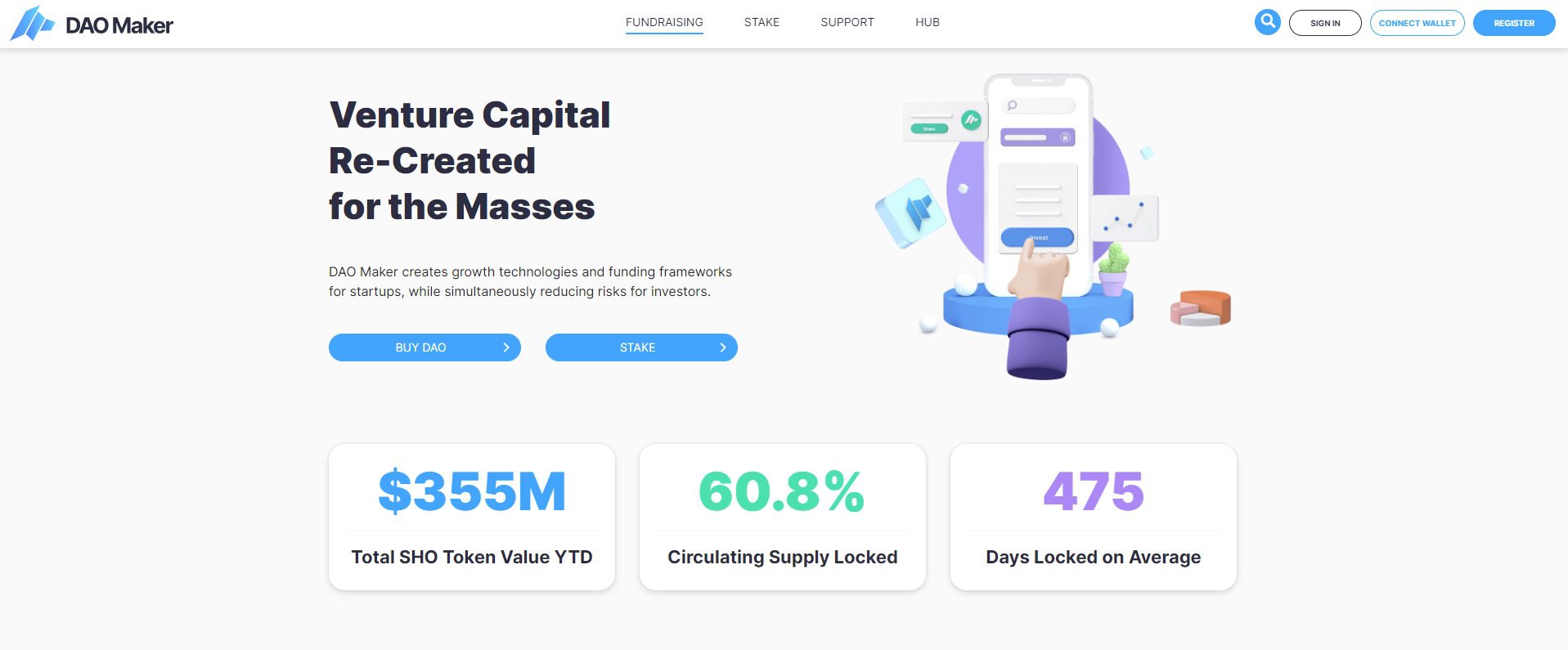This image features a detailed digital illustration with a rich background. At the forefront stands Dale Maker, accompanied by a blue dog. Prominently displayed text includes "DAO," which is capitalized, alongside underlined blue text labels such as "fundraising," "stake," "support," and "hub." A magnifying glass is positioned in front of a blue circle, suggesting a focus or search function.

Throughout the image, there are calls to action including "Sign In" and "Connect Wallet," albeit the latter is slightly small. Another key phrase, "Venture Capital Recreated for the Masses," indicates the theme or mission. Additional information related to DAOs and startups is scattered within the image.

At the bottom, three white rectangles contain critical data:
1. The first rectangle displays "355 million" with the "M" highlighted in blue.
2. The second rectangle details the "Total SHL Token Value YTD," with "YTD" in all caps, showing a circulating figure of "60.8%" in green.
3. The third rectangle notes an average value of "475 days" locked, indicated in purple. 

These elements collectively highlight financial metrics and operational details relevant to a DAO-focused venture capital initiative.